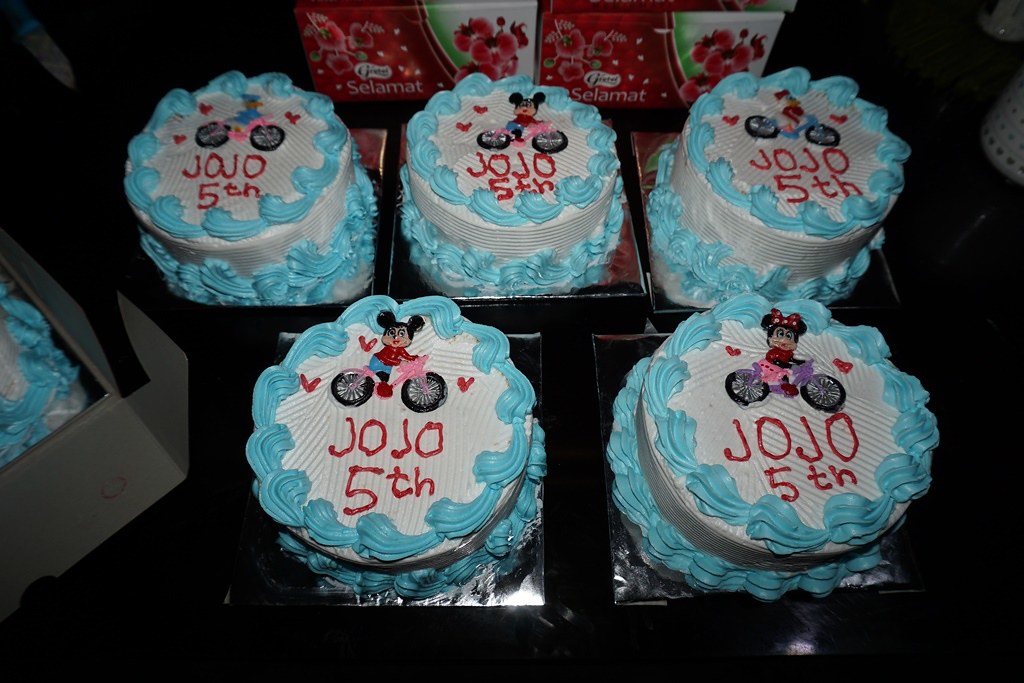This photograph features five small, round birthday cakes arranged on a black surface, each adorned with metallic foil squares. The cakes are decorated uniformly with a white frosting base and light blue swirls along the top edge and bottom. Each cake is inscribed with "JoJo 5th" in red piped letters. The cakes showcase different Disney characters riding bicycles. Specifically, one cake depicts Donald Duck on a pink bike, two feature Mickey Mouse—each on pink bikes, one displays Daisy Duck on a blue bike, and another shows Minnie Mouse with her characteristic red bow. To the left side of the photograph, there is the partially visible corner of a box containing a sixth cake. Additional elements in the background include two rectangular boxes, one red and one green, with floral designs and the word "Selamat." The environment around the cakes appears dark, enhancing the reflective surfaces and vibrant colors of the cakes.